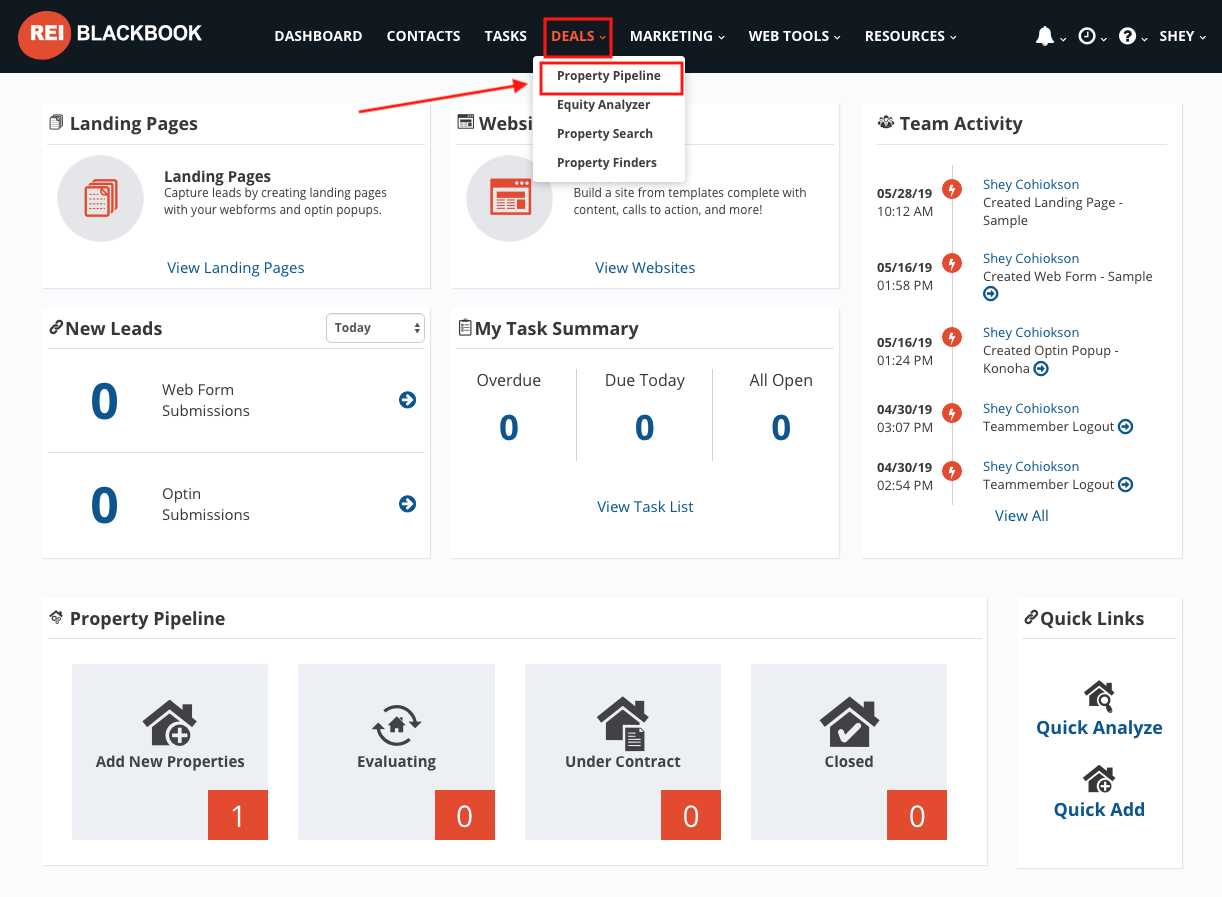This screenshot is taken from a website called Blackbook, a platform that appears to cater to real estate investment. Located at the top right corner of the interface is a black bar, while the top left corner displays a red logo with the letters "REI" in white font at its center. Next to the logo, the platform name "Blackbook" is also written in white font.

Below the logo, a navigation menu is available with several options, including Dashboard, Contacts, Tasks, Deals, Marketing, Web Tools, and Resources. The "Deals" option is currently selected and is highlighted with a red outline. The font for the selected option is in red. This selection reveals a drop-down menu with more choices: Property Pipeline, Equity Analyzer, Property Search, and Property Finders. "Property Pipeline" is pointed to by a red arrow and also enclosed in a red rectangle.

The main section of the website offers various features and information. On the left-hand side, "Landing Pages" are discussed, stating their purpose to capture leads through the creation of landing pages using web forms and optional pop-ups. On the right side of the main section, "Team Activity" displays some ongoing task information.

At the bottom of the page, there are four action buttons: "Add New Properties," "Evaluating," "Under Contract," and "Closed." In the bottom right corner, there are quick access links labeled "Quick Links," "Quick Analyze," and "Quick Add."